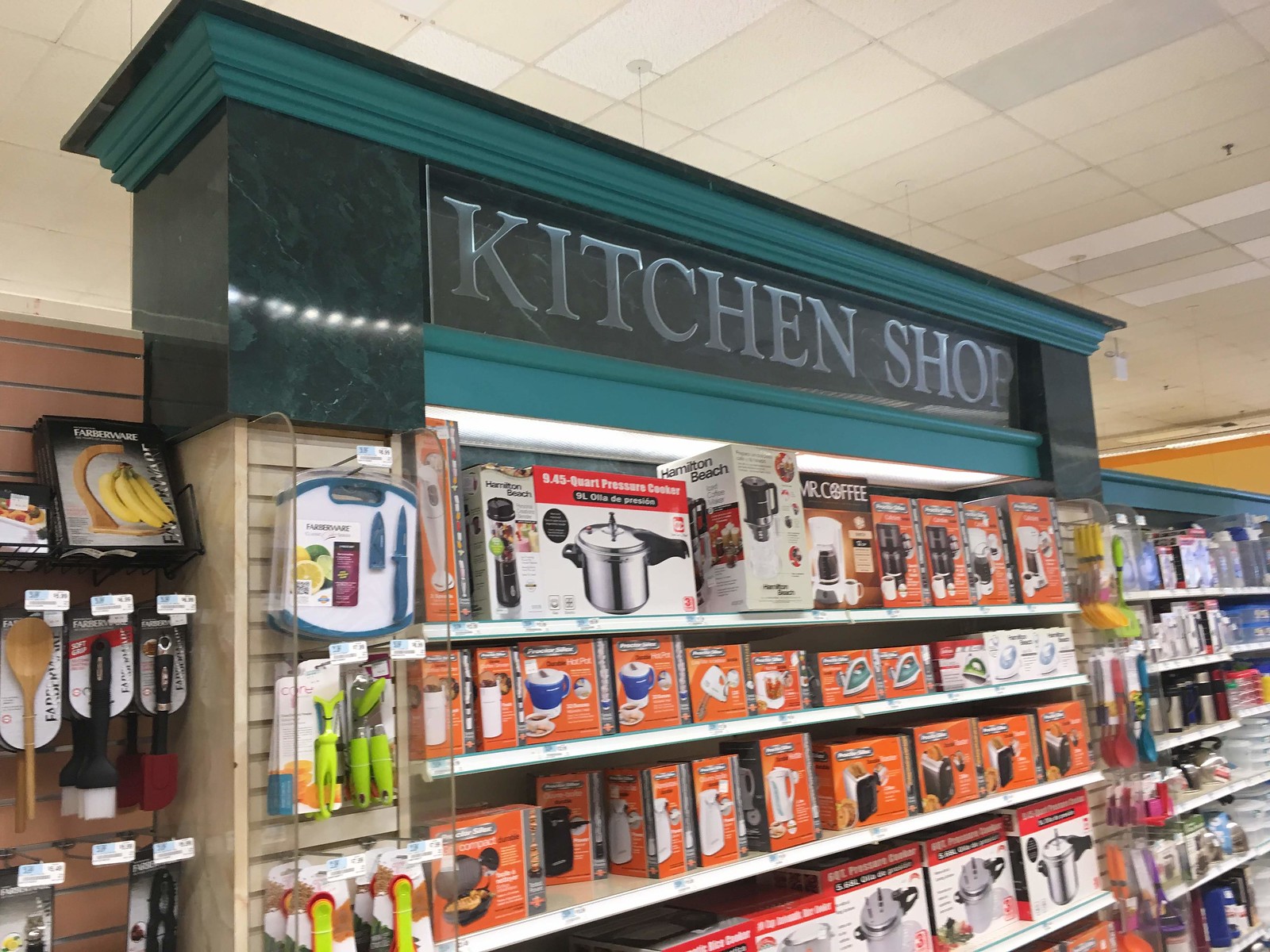This photograph captures a well-organized aisle within a store, specifically the kitchen section. Above the shelves, a sign reading "Kitchen Shop" is displayed against a dark green backdrop, accentuated with lighter green molding. Dominating the top shelf are large boxed items, including a 9-liter and a 4.45-quart stainless steel pressure cooker. Adjacent to these cookers is a chopping appliance from Hamilton Beach, followed by a coffee maker from the same brand. A Mr. Coffee white coffee pot encased in a black and brown box is positioned next to these. Various other coffee makers, with indistinguishable brand names, fill up the remaining top shelf space.

On the second shelf, we find white kitchen appliances from Proctor Silex, including a mixer and an iron. The shelf below hosts a stainless steel toaster from the same brand. The bottom shelf showcases larger, 5-quart stainless steel pressure cookers, each featuring black handles for easy use. The meticulous arrangement and diverse range of kitchen gadgets make this section a practical choice for shoppers seeking durable and reliable kitchen products.